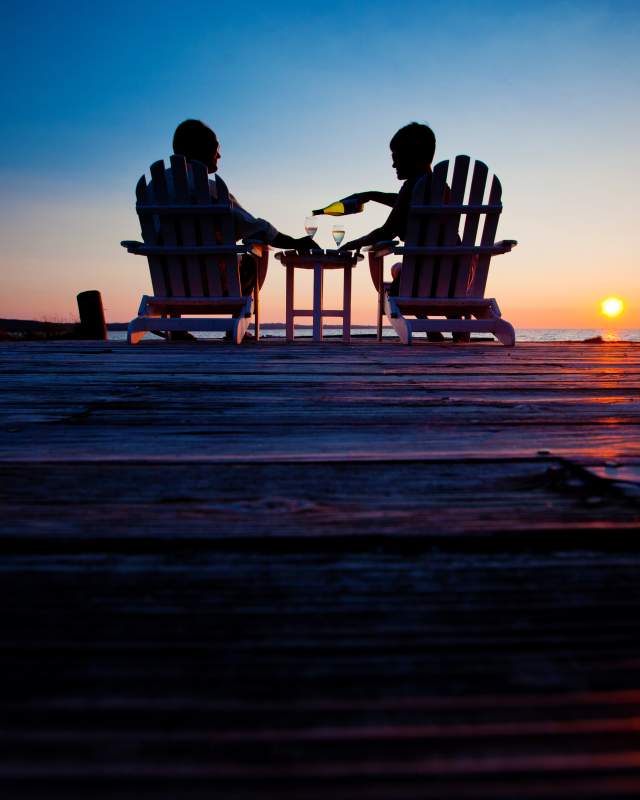In this evocative photograph taken just before sunset, two silhouetted figures are captured sitting on low wooden lawn chairs at the end of a wooden pier. The scene is bathed in the soft, fading light of dusk with most of the sky a deep dark blue, transitioning to hues of pink and orange near the horizon. Positioned with their backs to the viewer, the man on the left holds a wine glass while the woman on the right, turned slightly towards him, pours wine from a green bottle. Between them stands a small wooden table holding two wine glasses. The setting sun, a small yellow dot, hovers just above the horizon, casting a serene glow over the distant ocean visible beyond the edge of the pier. The overall scene is a perfect blend of tranquility and companionship, framed by the dimly lit sky and the gentle, reflective waters.